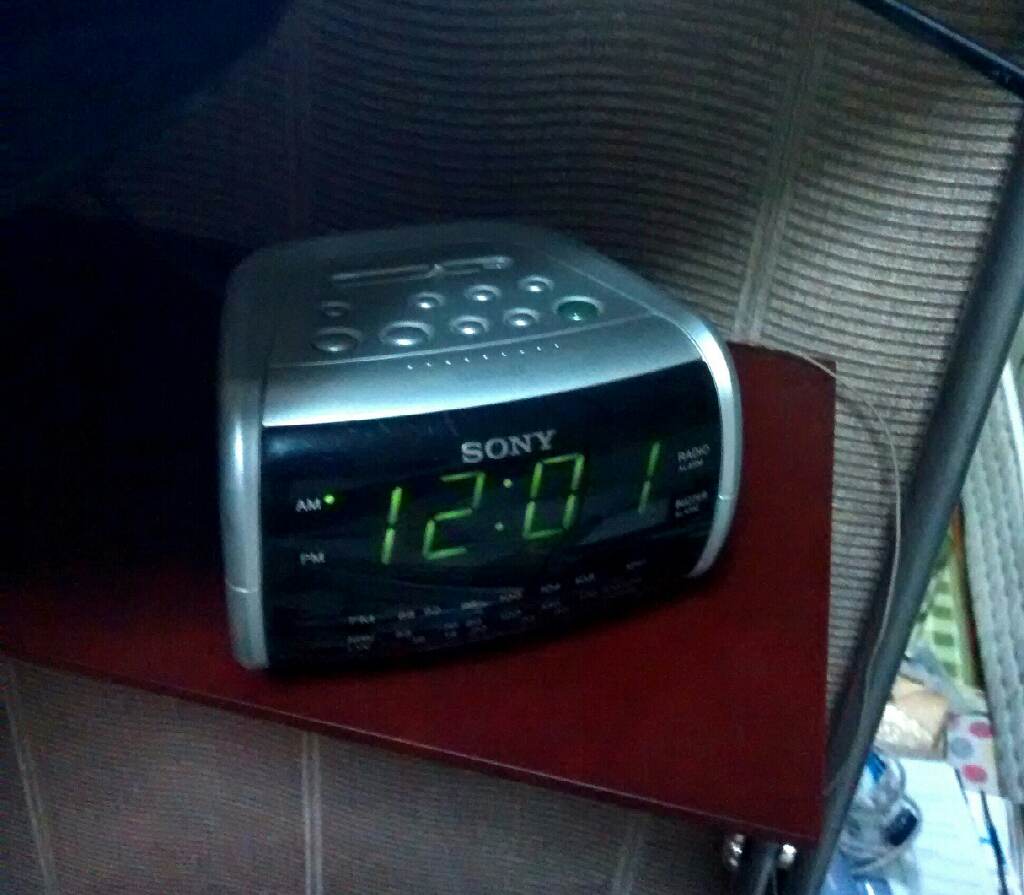The image depicts a bright and light-filled bedroom scene, centered around a Sony-branded alarm clock prominently displayed on a red, silver-legged dresser against a gray wall. This silver and black clock features a digital display reading "12:01 AM" in light yellowish-green digits. The display also includes radio settings, with a green light next to the AM indicator, and additional options at the bottom of the face. Numerous buttons are visible on the top of the clock, along with a clearly seen cord trailing off to the right. No people are present in the image, and a chair with fabric and black metal molding is discernible in the background.